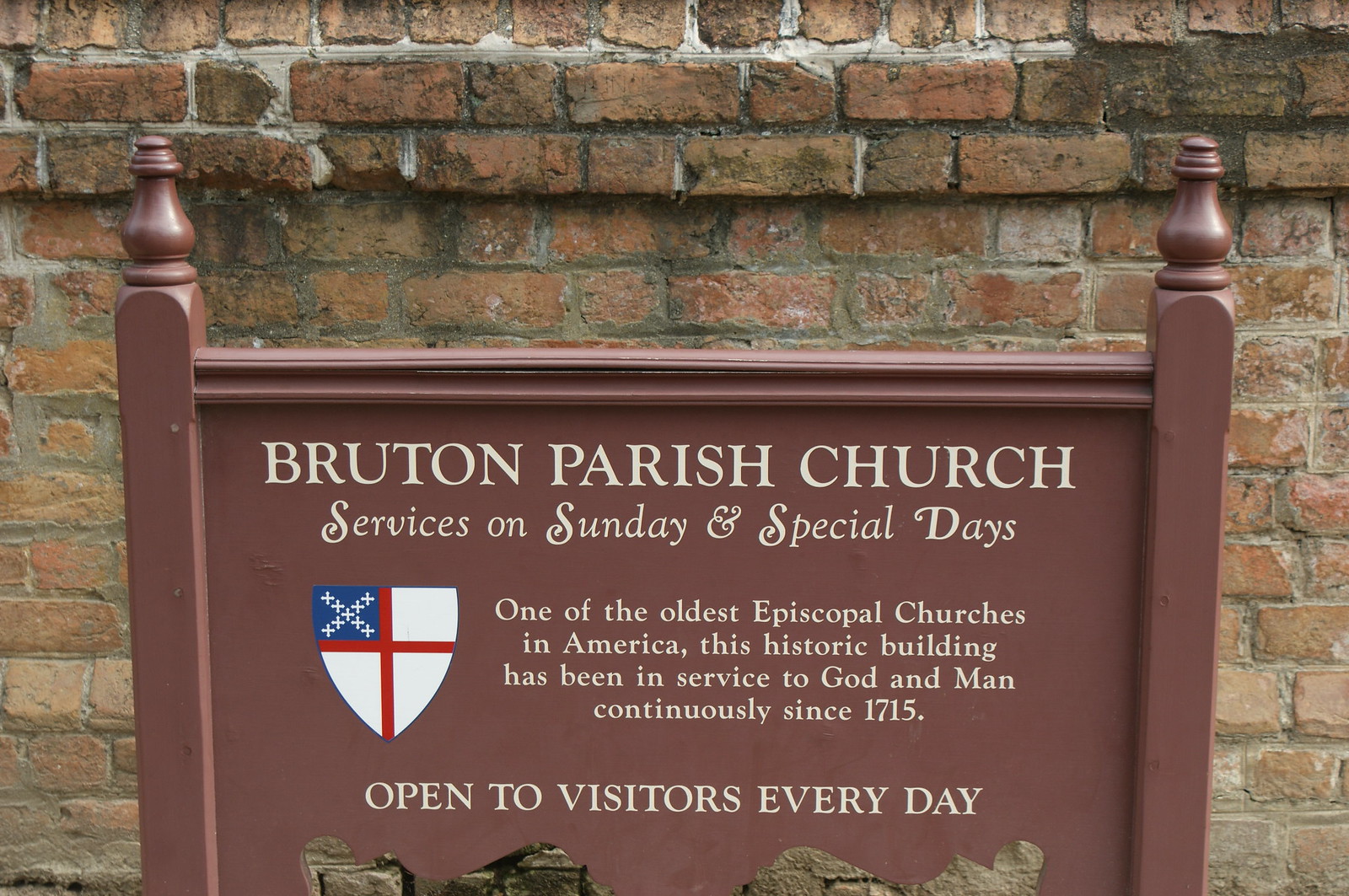This photograph captures an aged brick building with a historical wooden sign in front. The sign, which has a medium to burgundy-brown hue, features ornamental knobs on its sideboards, blending rustic charm with antiquity. The sign reads, in white letters: "Bruton Parish Church, services on Sunday and special days. One of the oldest Episcopal churches in America. This historic building has been in service to God and man continuously since 1715. Open to visitors every day." Below the text, there is a distinguished emblem of the Episcopal Church, presented as a white shield with a red cross intersecting it. The upper left quadrant of the shield is blue, with a white X composed of smaller crosses. This ancient church, likely situated in a historic district that attracts tourists, stands as a testament to its continuous service and rich heritage.